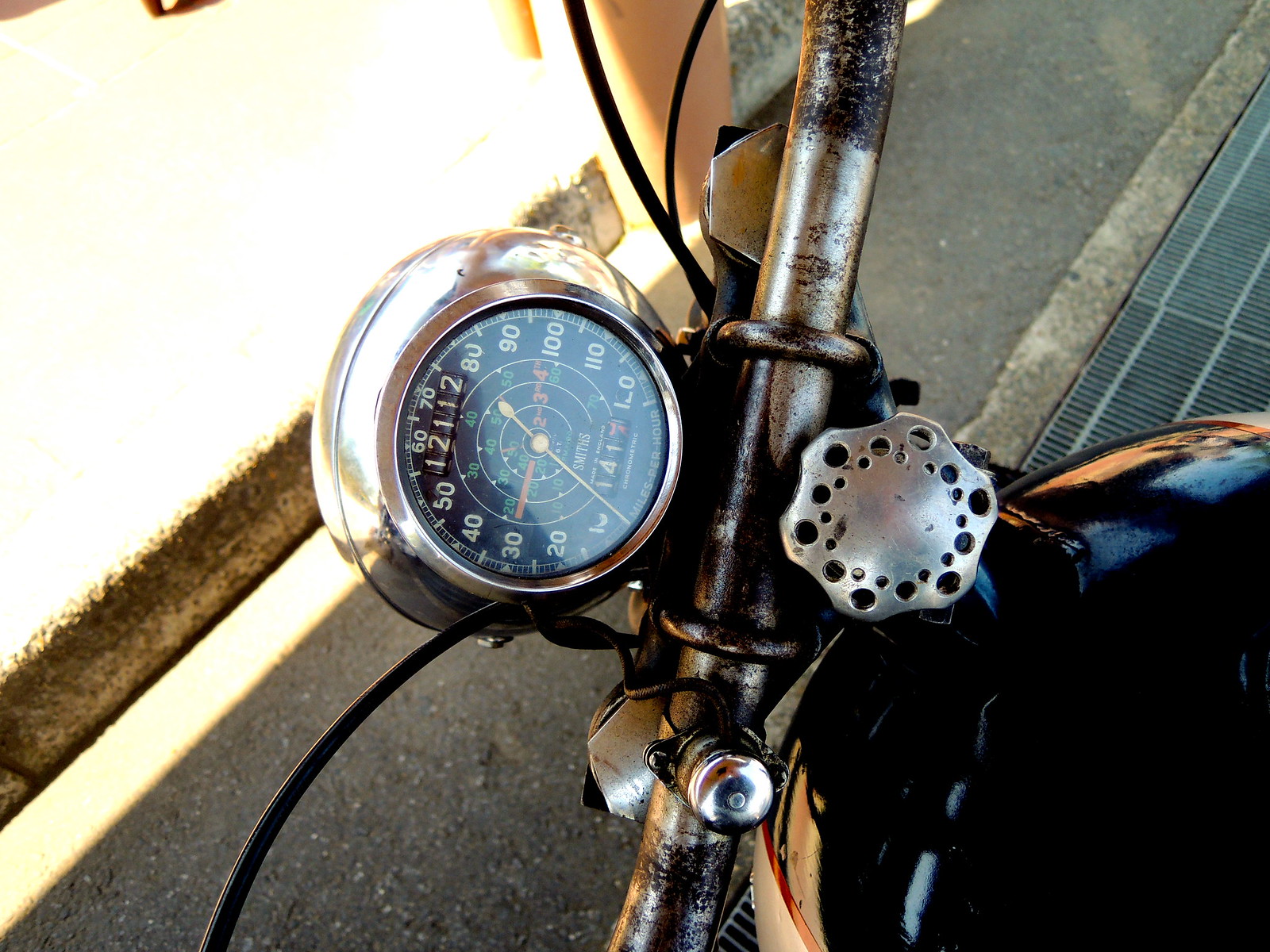In this close-up image, we are presented with a detailed view of a vintage motorcycle's handlebars and speedometer. The motorcycle exudes an aged charm, with significant rust adorning the handlebars and speedometer, which is encased in a round, shiny metal housing centrally positioned on the handlebar. The speedometer’s casing, despite the rust, still gleams slightly, adding a touch of nostalgia to the scene. Below the handlebars, a glimpse of the motorcycle’s shiny fuel tank is visible, further emphasizing its classic design. The background reveals an asphalt surface, indicating the motorcycle is parked on a metal drainage grid. Adjacent to this, there is a rusted door on the ground, contributing to the overall rustic ambiance of the setting. Every detail in this photograph accentuates the motorcycle’s vintage essence and long history.